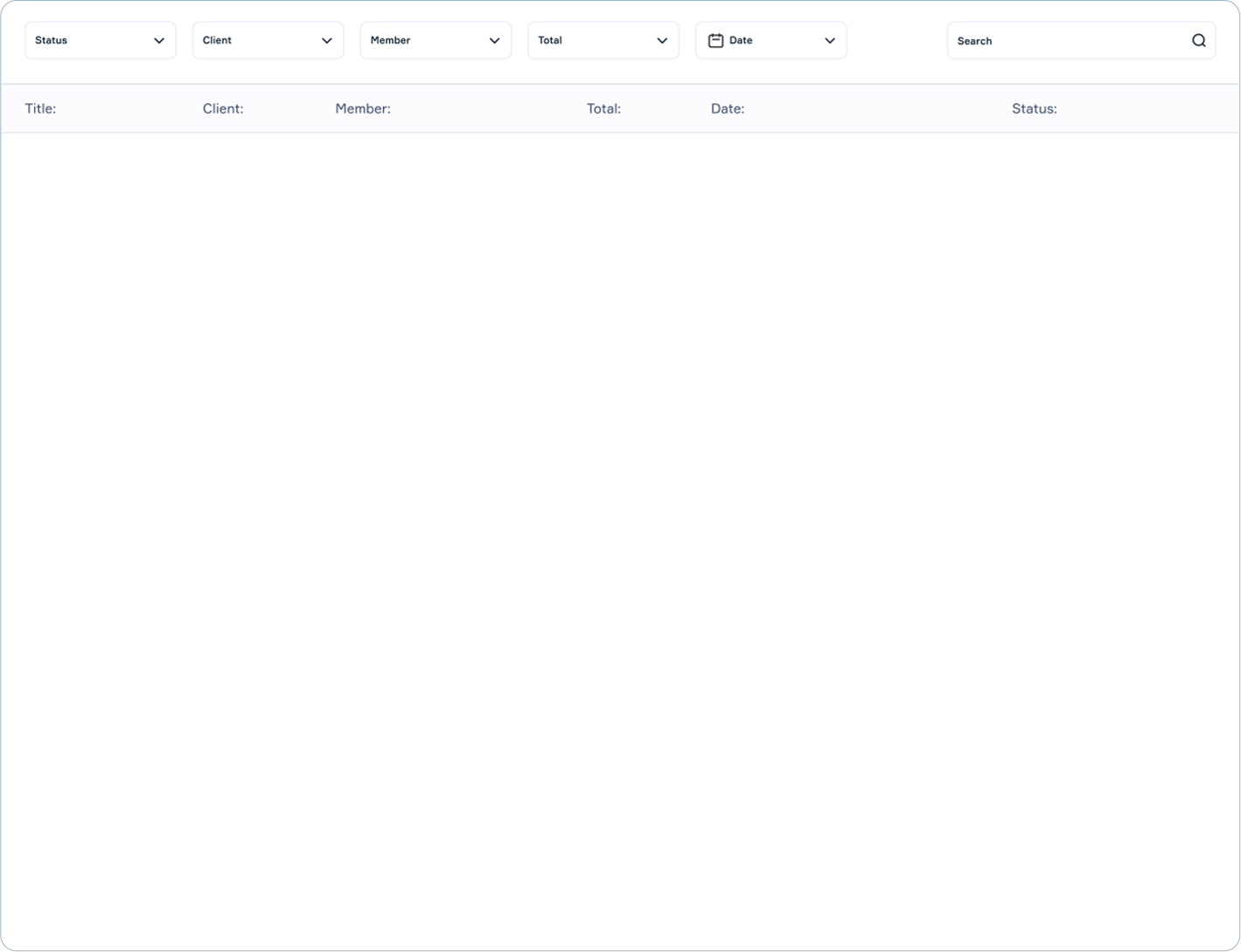The image depicts a simplistic and minimalistic website layout devoid of any header or title. The primary structure consists of several horizontally arranged categories from left to right. The first category, labeled "Status," is presented in a white box and is accompanied by a drop-down menu. Adjacent to it are the categories "Client," "Member," and "Total," each with their own drop-down menus. Further along is the "Date" category, also featuring a drop-down menu, followed by a nondescript symbol and a search bar.

Beneath these top-level categories lies a light blue bar with repetitive labels: "Title," "Client," "Member," "Total," "Date," and "Status," though no additional content is provided below this bar.

The website's overall aesthetic is characterized by a white background framed by a light gray border. Each of the category boxes at the top is outlined with light blue, further detailed with double gray lines—one at the top and another at the bottom. The absence of any identifiable purpose, branding, or contextual information renders the website exceedingly generic and plain.